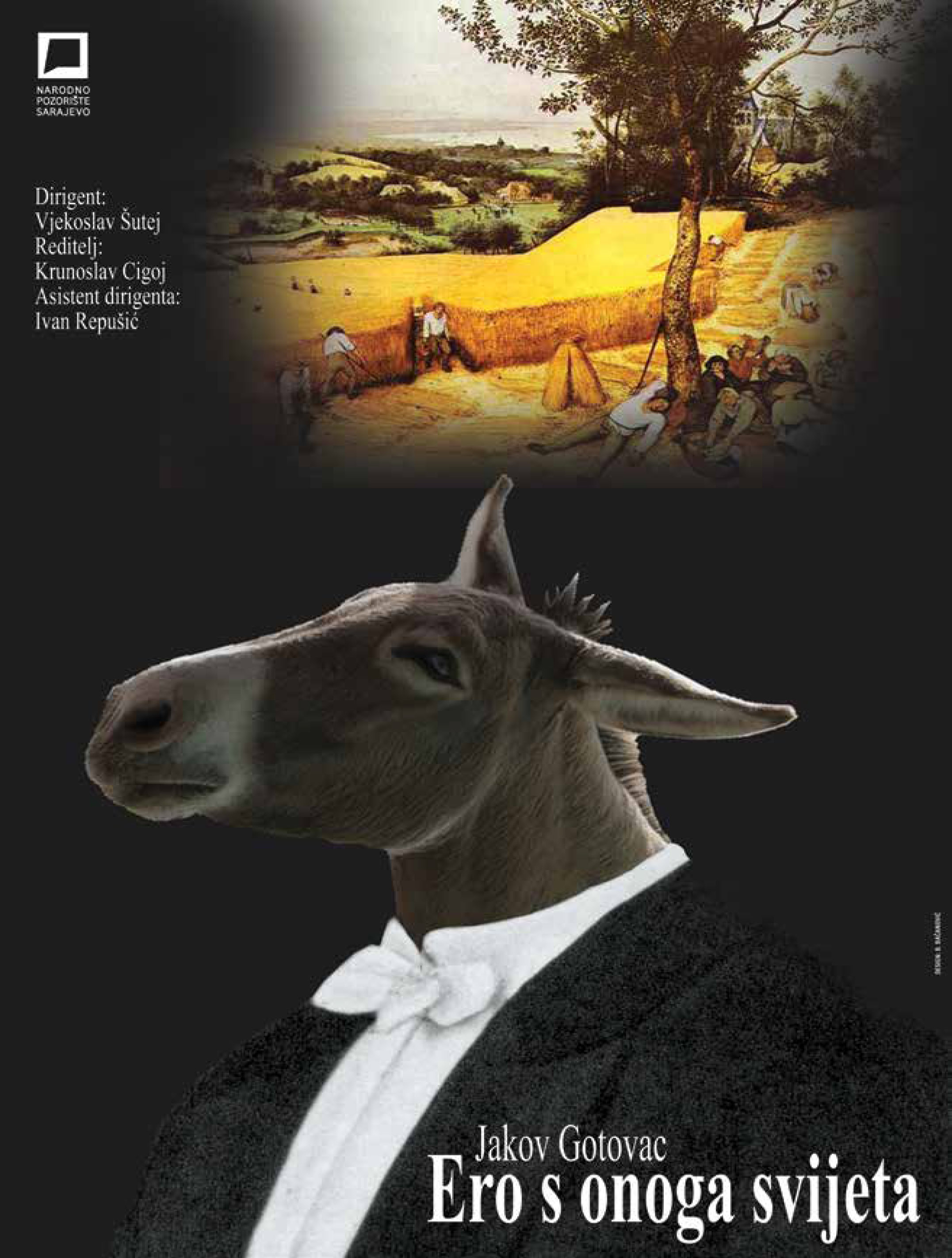The poster presents a surreal composition divided into two distinct sections. The top part displays a vibrant painting of golden fields with laborers actively working and others resting, all set against a picturesque backdrop of a green valley, distant houses, and a solitary tree. Detailed elements include women and men harvesting hay, a worker arranging food, and another lying down near the field. The bottom part prominently features the head of a gray donkey seamlessly superimposed onto the torso of a man dressed in a formal black coat, white shirt, and bowtie, against a black background. Additionally, white text in a foreign language adorns the upper left corner and the bottom section of the poster, with the words "Jakov Godovac Eros Onoga Svijeta." The overall style of the poster is Surrealism, blending realistic pastoral scenes with fantastical elements.